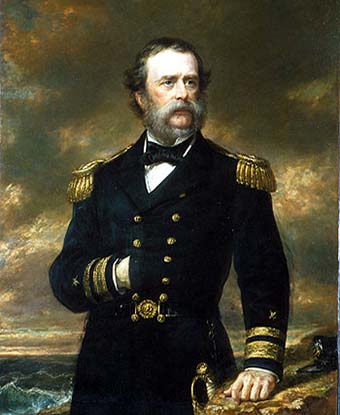The image depicts an older, distinguished white military officer, possibly from the navy, dressed in a traditional dark blue uniform adorned with extensive gold accents. His uniform includes two rows of golden buttons down the front, gold tassels on his shoulders, and gold bands around his cuffs. He is wearing a black bow tie over a white shirt, and a belt with a prominent gold buckle at his waist. The officer has a notable long grayish beard and mustache and dark brown hair. His right hand is tucked inside his jacket, reminiscent of Napoleon's famous pose, while his left hand rests on a rock. A sword with a gold handle is visible on the left part of his leg. The background reveals a stormy, cloudy sky with light peeking through, and white-capped ocean waves below, providing a dramatic and classic portrait setting.